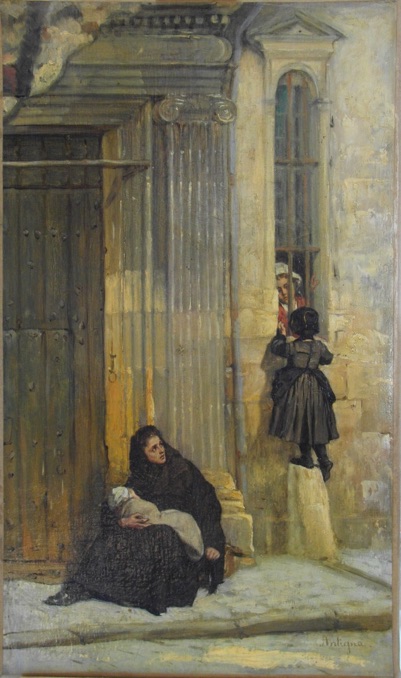In this evocative painting reminiscent of the muted earth tones and darker pigments typical of the 1800s, we see a captivating street scene. A woman dressed head-to-toe in black sits on a stone sidewalk before a modest, roughly 10-foot-tall wooden door, which may serve as the entrance to an old church. The door is situated on the left side of the composition. The woman, who has a fair complexion, sits with her back against a pillar beside the door, gazing over her shoulder toward the left, her head angled at about 330 degrees.

Cradling an infant swathed in a tan or beige blanket that conceals much of the child’s form, the woman presents a serene yet somber figure. To her right, a young girl, also clad in a long black dress, stands elevated on a decorative ledge or piece of stonework. Her back faces the viewer as she looks into a narrow, barred, oval window. Behind the bars of this window, a woman in a white bonnet and red dress peers out, creating a focal point of interaction within the painting.

The scene is set against a backdrop of weathered stone walls, with hues of gray, beige, and touches of blue, reflecting a medieval atmosphere. The heavy wooden door and the stone elements around it emphasize the age and solemnity of the setting, evoking the charm of an antique painting that might be found in an art book from the 1800s.